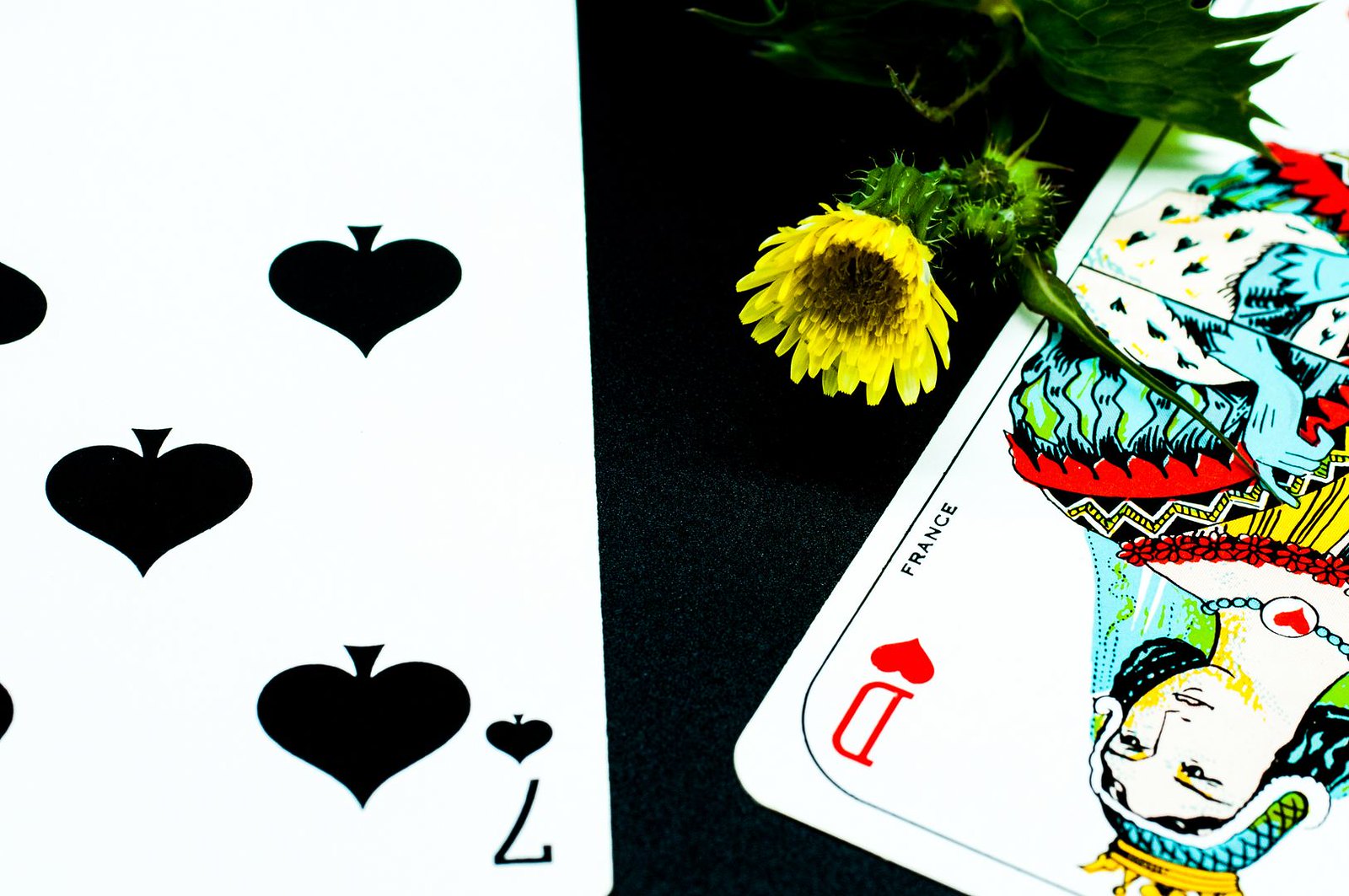In the image, there are two playing cards displayed prominently. The first card is the seven of clubs, with the clubs arranged in an inverted fashion, resembling small black hearts with a stem emerging from the bottom, similar to an apple. When viewed upside down, these shapes transform back into traditional clubs. Adjacent to this is a card featuring the queen of diamonds. The card is adorned with the word "France," suggesting it could be either a playing card or a tarot card. The queen depicted wears an ornate crown and a necklace, which features a heart emblem, making her reminiscent of the queen of hearts motif. Atop this card lies a sunflower, or possibly a cornflower, with one of its leaves draped across the card's surface. The vivid yellow petals of the flower are clearly visible, and the stem, accompanied by additional leaves, stretches across the queen's image.